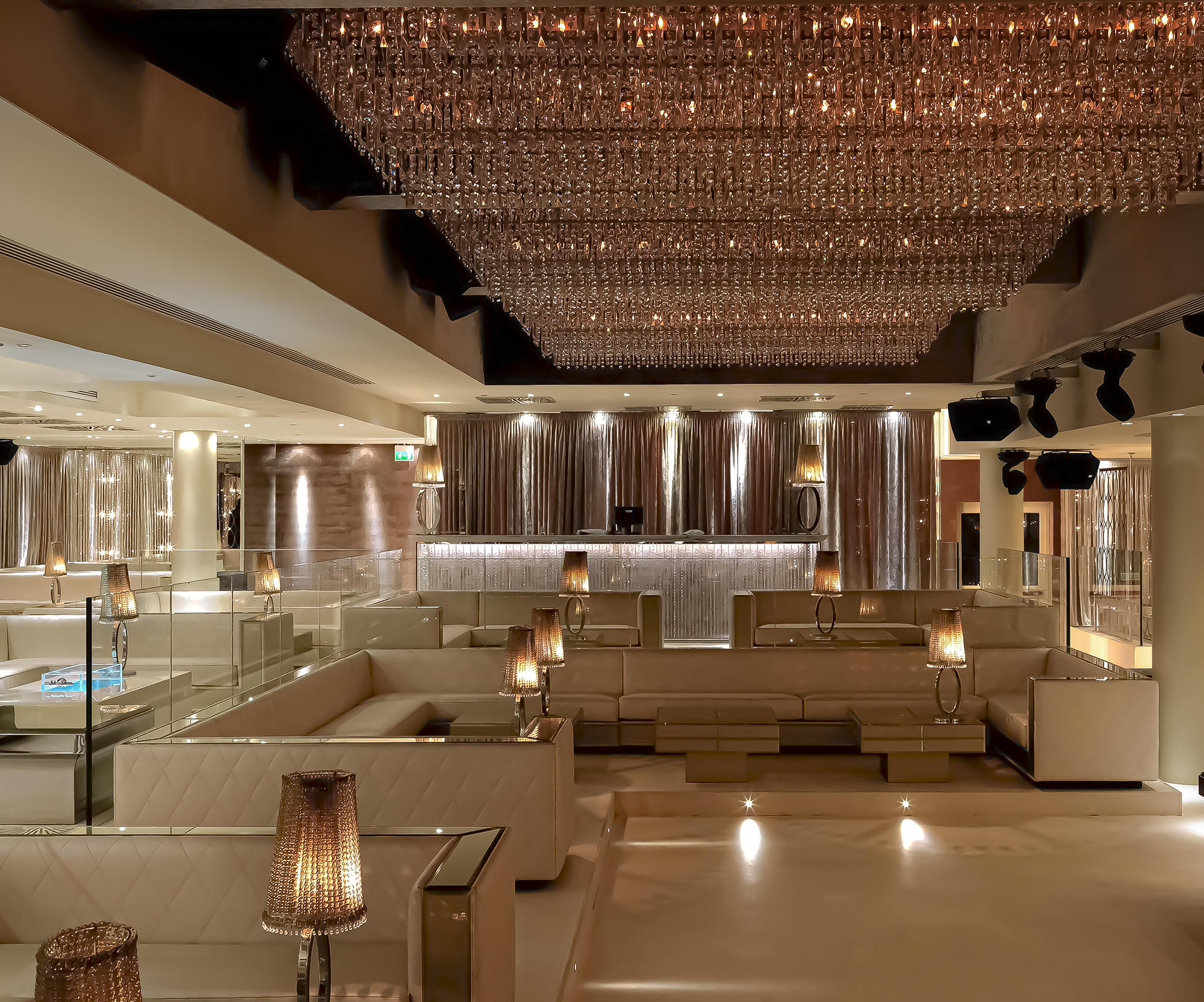This image showcases an opulent, high-end lounge area predominantly adorned in beige tones. The space is furnished with an array of sectional and standalone sofas, characterized by their rigid, square shapes and strong lines. A prominent L-shaped sectional sofa takes center stage, accompanied by two additional sofas in the background and a partial view of another similarly styled sofa in the foreground. The lounge is further accentuated by several slim, stylish table lamps perched on small tables in front of the sectional sofa. The ceiling features an intricate design with glass elements and chandeliers, enhancing the elegance and luxurious feel of the space. The overall atmosphere is one of refined sophistication and upscale comfort, perfectly blending modern design with timeless elegance.